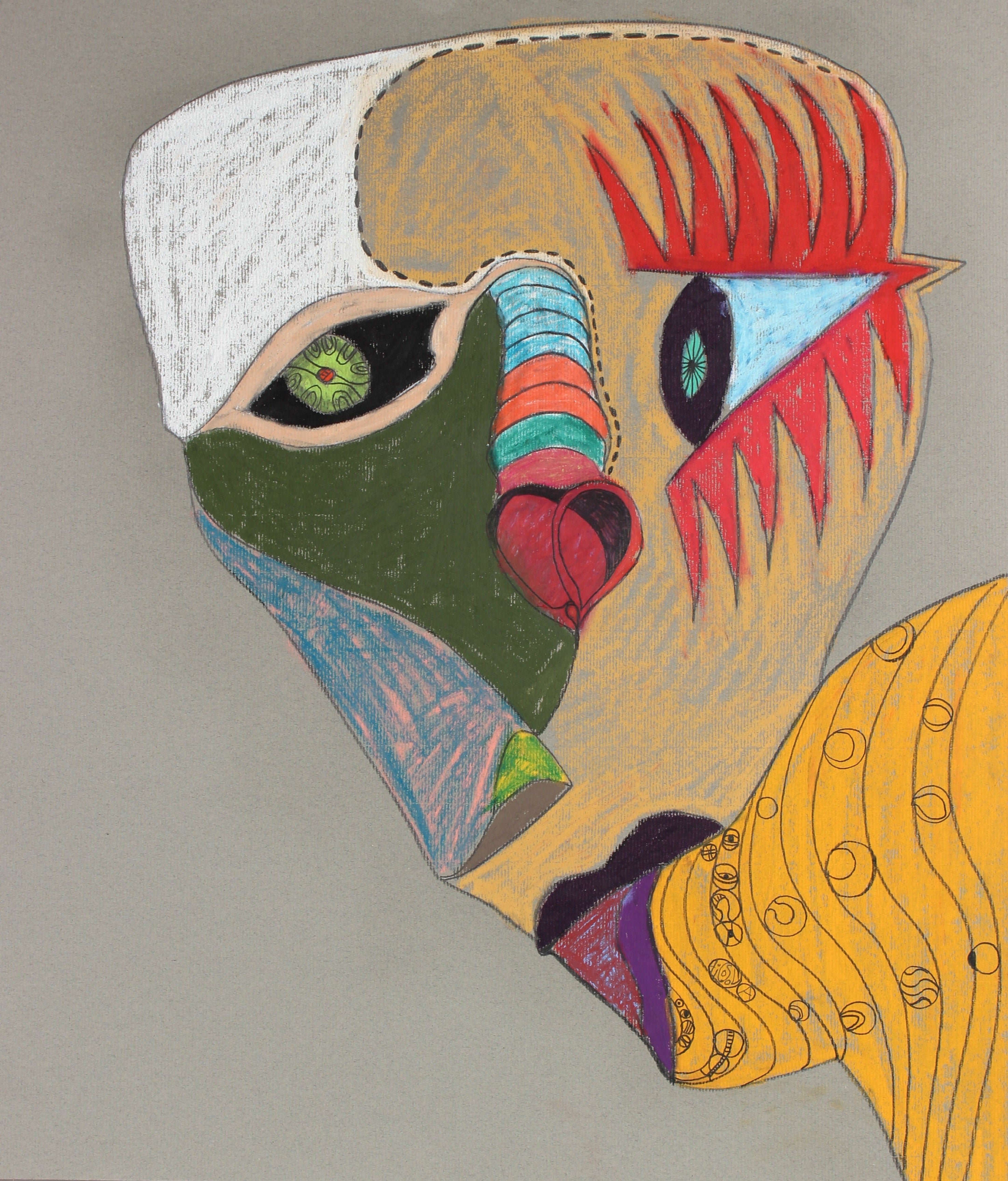This abstract artwork, reminiscent of a Picasso-style painting, features a perplexing composition on a grey, chalk-like background. The central figure, occupying a substantial portion of the image, has a bulbous, asymmetrically sectioned head resembling an upside-down triangle, though rounded. The face is divided into various colorful, wavy sections: white in the left corner, orange extending down the right side to the chin, a green patch beneath the white, and a blue section on the side. 

The left eye is circular, outlined in peach with a black sclera, a yellow iris featuring double ovals, and a red pupil. The right eye is distinctly 3D and cone-shaped, with a white triangle and a black core containing a blue center. Prominent, exaggerated red eyelashes frame this right eye, adding to its striking appearance.

The nose is an unusual, segmented tube with blue and red stripes running vertically. A heart-shaped mouth displays an open black shadow and a red tongue on one side, creating the appearance of a looped string, further emphasizing the heart shape.

Beneath the head, the figure seems to transition into an animal-like form, with an orange segment that extends off to the side like the beginning of an animal's body. Additionally, the figure wears what appears to be a gold shirt with a purple cuff adorned with intricate curlicue designs, adding a touch of surreal elegance to the otherwise bewildering and compelling image.